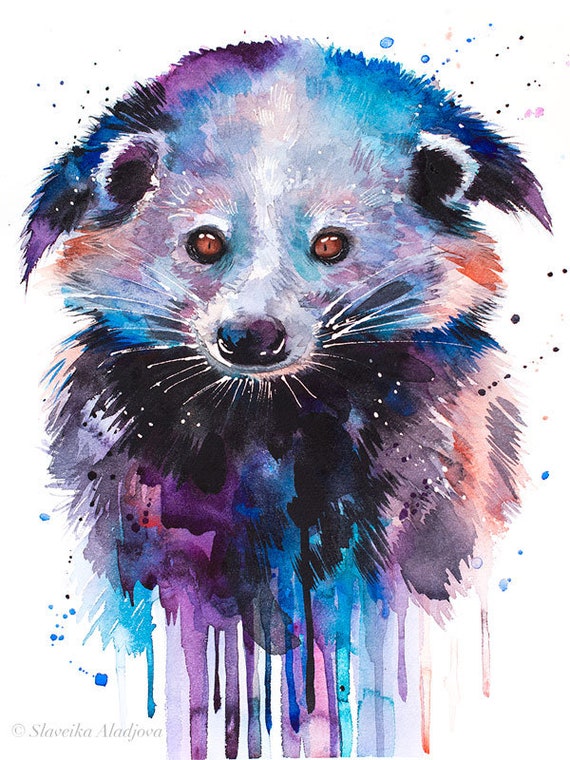This watercolor painting features a whimsical, fox-like creature against a stark white background. The creature’s face, rendered in vivid detail, showcases a pointy black nose, white whiskers, and expressive brown eyes surrounded by hints of orange and black eyeshadowing. Its ears are a striking mix of white, black, and purple, adding to the unique aesthetic. The fur on its head is an eclectic blend of blue, purple, and black hues, with splashes of orange. Below the meticulously detailed head, the body transforms into an abstract, undefined round shape swirled with shades of blue, black, lilac, pink, and teal, giving the impression of colorful paint blobs and drips. These drips flow downward, adding a dynamic, almost melting effect to the piece. The artist's delicate control over the medium is evident in the intentional paint splatters and drips extending from the creature, mimicking classic mall posters' stylized imagery. The bottom left corner bears the artist's watermark, reading "Slavica Eladjova."